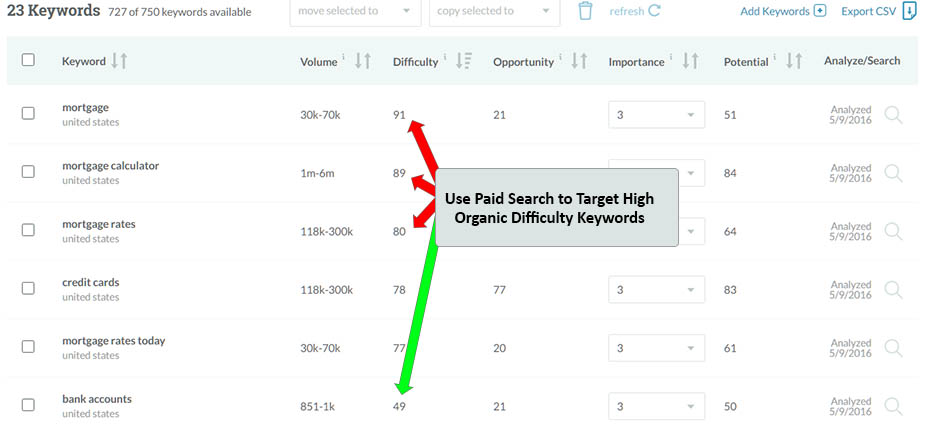A comprehensive dashboard overview highlights opportunities for the user to increase traffic. In the upper left, 23 primary keywords are displayed, alongside a count of 727 out of 750 possible keywords. The interface includes options to move or copy selected keywords, a trash can icon for deletion, a refresh button, an 'Add Keywords' button, and an option to export data as a CSV file.

The dashboard headers are categorized as follows: Keyword, Volume, Difficulty, Opportunity, Importance, Potential, Analyze, and Search. Each header features sortable arrows, and the left-hand side contains checkboxes for each category. The visible data entries include keywords such as "mortgage," "mortgage calculator," "mortgage rates," "credit cards," and "bank accounts," all specific to the United States market.

Important metrics are visually indicated with red and green arrows, suggesting strategic focus on high organic difficulty keywords to boost traffic. Difficulty ratings show that "mortgage" has a rating of 91, "mortgage calculator" is 89, "mortgage rates" is 82, and "bank accounts" is 49, each accompanied by directional indicators. 

Volume metrics highlight significant search frequencies, with "mortgage rates" and "credit cards" each having an estimated volume range of 118,000 to 300,000 searches.